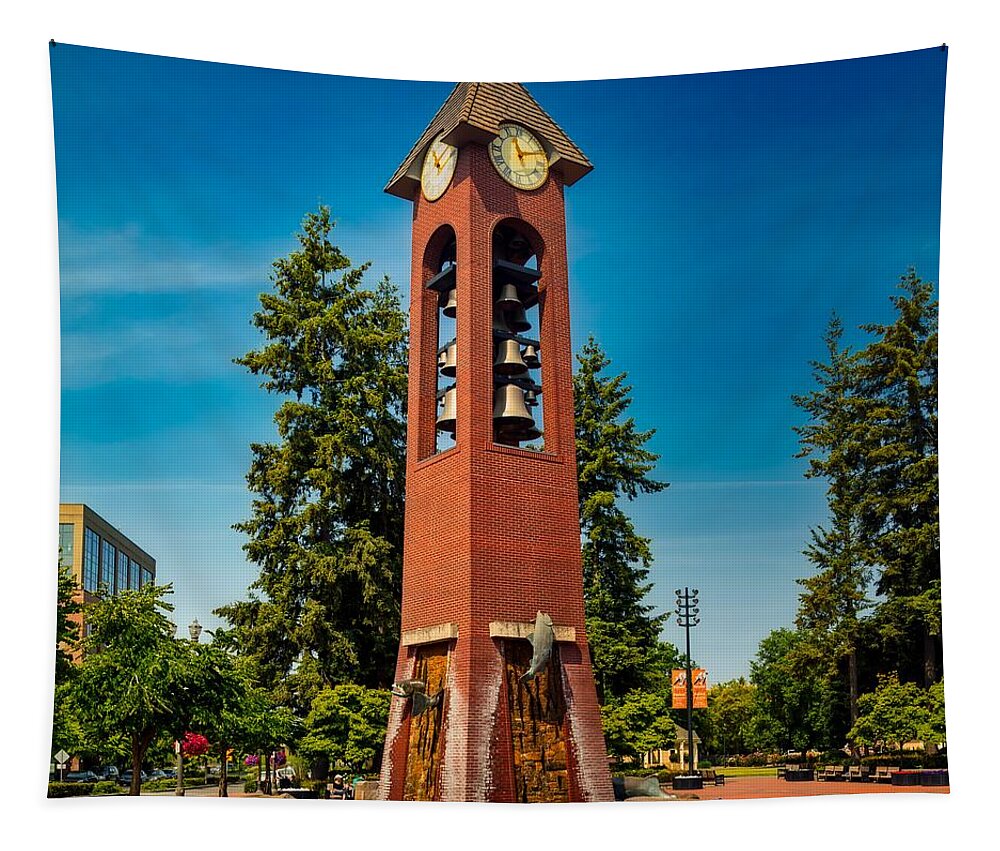This square-format, color photograph captures a striking bell tower standing prominently in the middle of a town square, or plaza. The tower, constructed of red and brown brick, stands about the height of a three-story building and features a design that flares out slightly at the base, adorned with wood insets and decorative fish sculptures. Each of the tower's four sides showcases arched openings near the top, containing three tiers of bells, totaling 12 bells in all. Above these arches, a pointed, shingled roof supports four round clocks, one on each side. The scene is set on a clear, blue day with only a faint hint of cloud haze, and the tower is surrounded by trees, manicured walkways, and brick buildings. Cars can be seen beneath the trees, and to the left, a larger building and a church are visible, while the right side features additional lighting and buildings. The harmonious blend of natural and architectural elements creates a picturesque and serene atmosphere, perfect for outdoor relaxation.